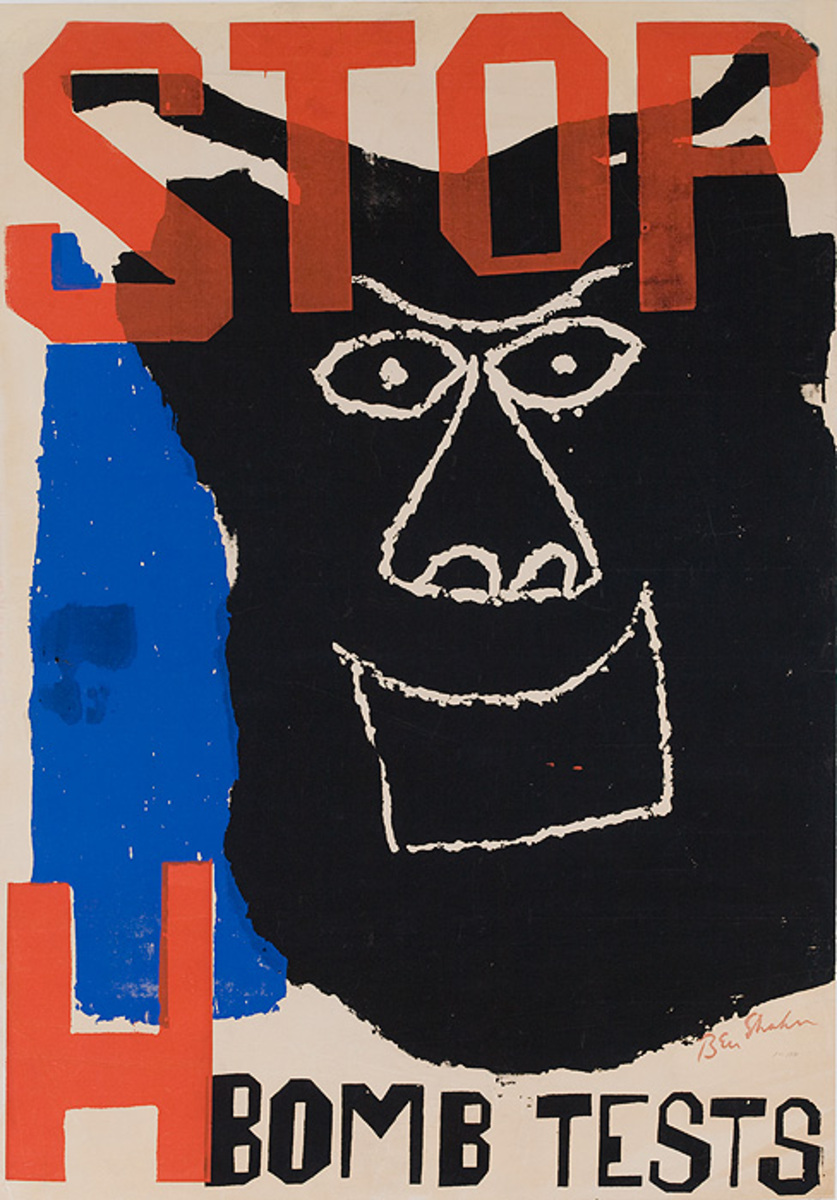The image is a detailed, hand-drawn painting set against a cream-colored background with prominent red capital letters at the top that read "STOP H BOMB TESTS." At the bottom left, the text continues with "H bomb tests," completing the anti-nuclear message. Dominating the foreground is a large, black, cartoonish head that appears both human and animalistic, with expressive eyes, a prominent nose, and a wide mouth. The head is ambiguously rendered, suggesting it might be a gorilla because of its black color and shape. To the left of this face, there's a vertical blue stripe, reminiscent of a pillow or similar object. The lower part of the painting includes an artist's signature, reading "Ben S," though the last name is not fully legible. This powerful imagery and bold text serve as a stark statement against the testing of hydrogen bombs.